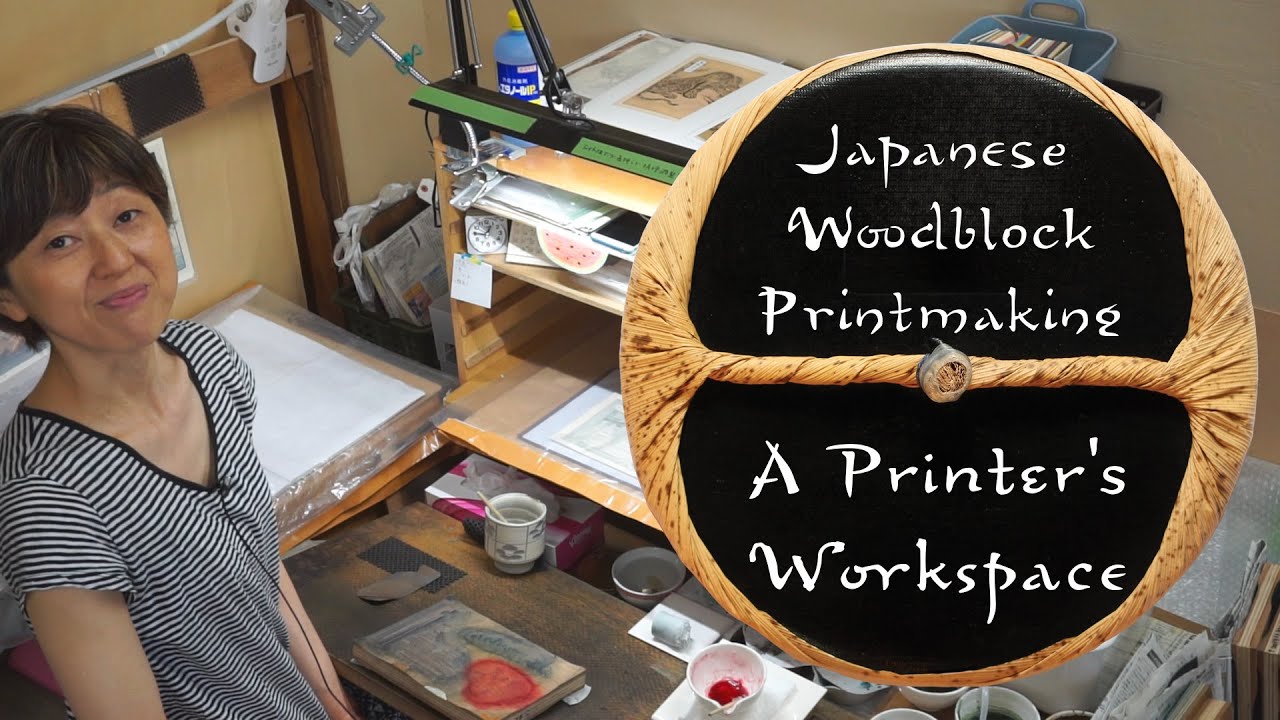The photograph and advertisement showcase a Japanese woodblock printmaking service, featuring a printer's workshop. In the image, a Japanese woman with short, ear-length black hair smiles at the camera. She's dressed in a black and white, horizontally striped V-neck short-sleeve shirt. The left side of the image is dominated by her presence, while the right side reveals her workspace. 

The workshop includes a well-used, darker wooden desk cluttered with various supplies like paints, paintbrushes, cups, a book, and numerous white papers. Some of the paint supplies, including red paint, are visible, enhancing the vibrant, creative environment. The wall behind her workspace is light brown or beige, contributing to the warm, rustic feel of the room.

To the right of the image is the logo, featuring white text on a black background with brown accents. The logo reads "Japanese woodblock printmaking, a printer's workshop" and is designed within an elongated circular shape, twisted in the middle, giving a wooden, paper-like appearance with darker brown spots for added texture. The photograph effectively promotes the traditional craft and inviting atmosphere of the printmaking service.